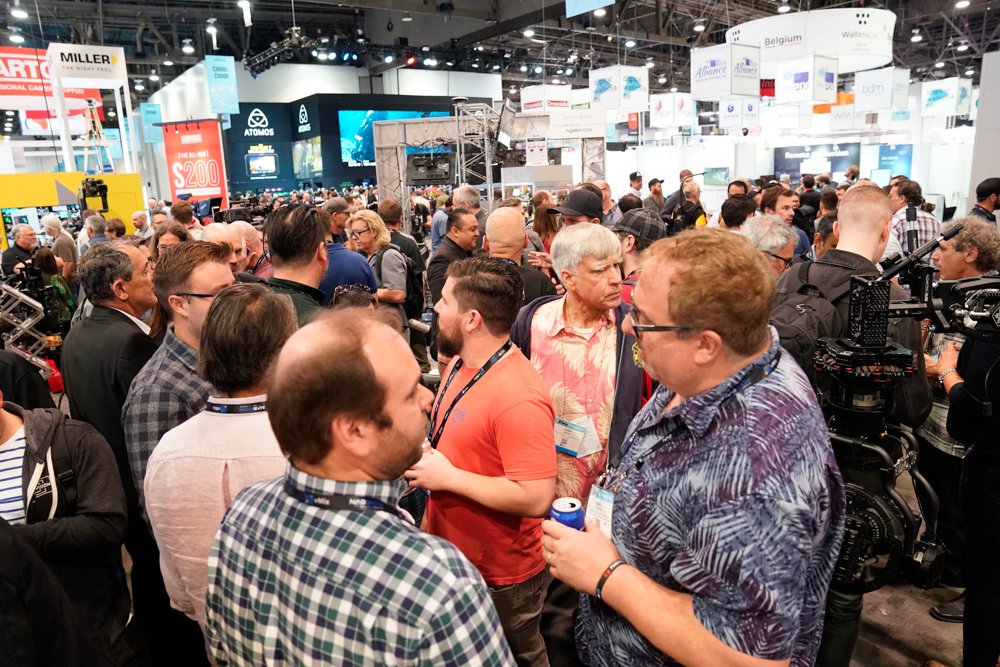This photograph captures the bustling atmosphere of an indoor convention, featuring a diverse crowd predominantly composed of adult white males. The convention space is expansive and well-lit, with the ceiling obscured by grey bars and rafters, possibly indicative of an unfinished room or a large community center. Rows of bright lights dangle overhead, contributing to the vibrant energy of the scene.

In the background, a series of boxy, square-shaped advertisements and brand displays stretch across the upper part of the image, made from materials that suggest they can be easily assembled and disassembled. Prominent among these is a banner for "Miller" in bold black capital letters with a yellow emblem beneath it. Another red and white banner reads "ARTO," bordered in white, and a dark blue banner with a white, upside-down heart-shaped logo. These displays seem to illuminate, adding to the vivid setting.

The foreground is dense with attendees, all casually dressed. Two men on the bottom left sport blue checked plaid shirts, both with sandy blond hair, separated by another man. Most individuals wear grey lanyards with white text and a blue emblem, hinting at a unified theme or organization. One notable figure on the right wears a conspicuous blue, purple, and light blue button-up shirt adorned with palm fronds, holding a Pepsi can and wearing spectacles and a wristband. Behind him, a slightly older man with gray hair and a red shirt also decorated in palm fronds looks to the right.

Interspersed within the crowd are people holding drinks, backpacks, and media equipment, all contributing to the dynamic and engaging environment. One potential female attendee can be seen on the far left in a black jacket with a white and blue vertically striped shirt, blending into the mix of individuals who fade into the background of the busy convention floor. The setting evokes a contemporary feel, though the styles visible leave open the possibility of a scene from as early as the 1980s.